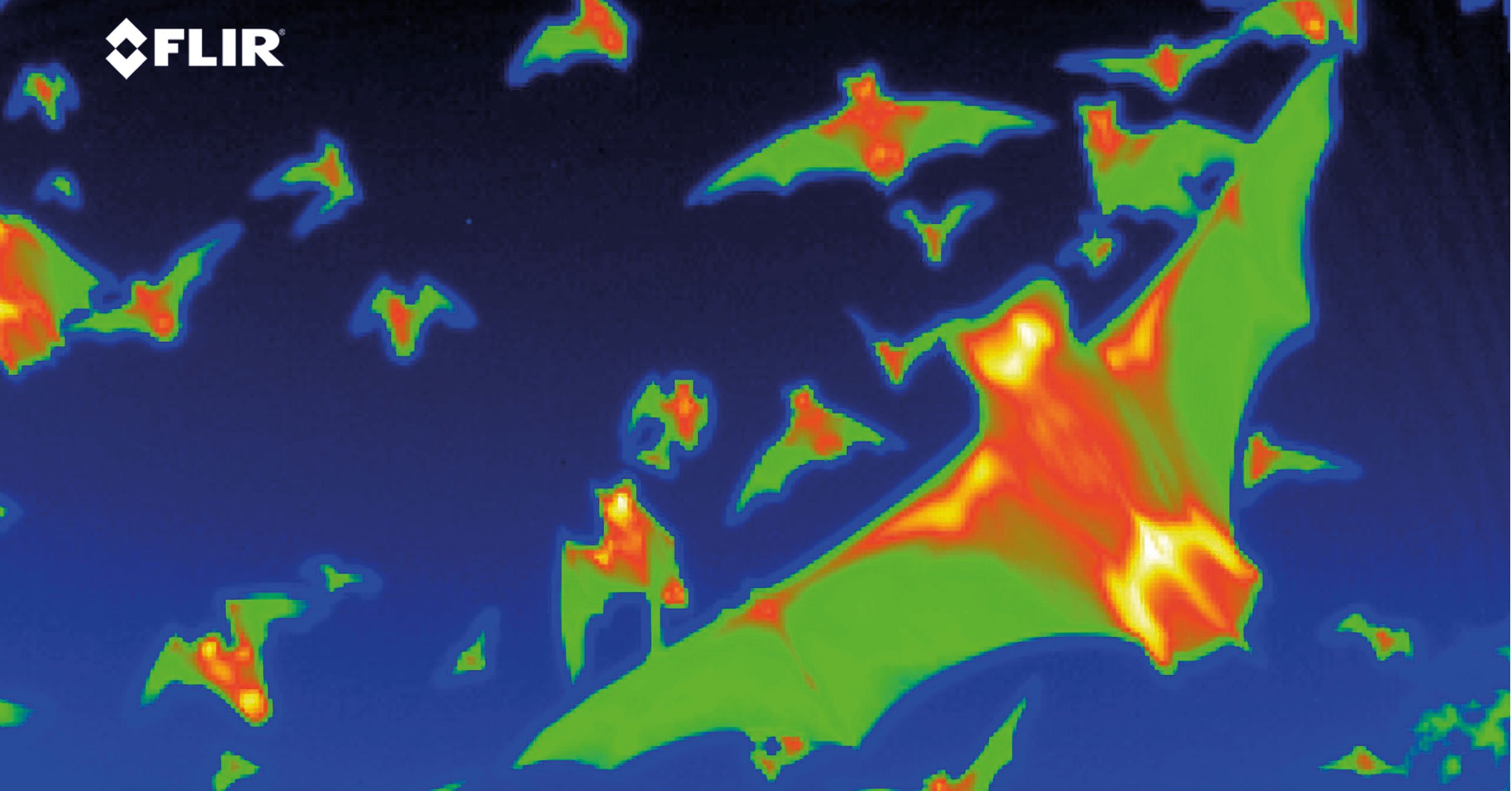The image is a thermal photograph capturing a swarm of bats in flight at night. The backdrop of the photo transitions from nearly black at the top to a lighter, yet still dark, blue as it goes downward. FLIR’s logo, featuring a pair of opposing arrow-like symbols, appears in white in the upper left-hand corner.

The bats are visualized in vibrant thermal colors. Their wings exhibit cooler tones of green, while their bodies show warmer hues of yellow, orange, and red, indicating higher heat concentrations in those areas. Numerous bats populate the scene, ranging in size and distance from the viewer. The one nearest to the camera is prominently displayed, offering a clear view of its heat signature. In contrast, other bats are scattered throughout the background, some barely visible.

The overall composition emphasizes the varying heat intensities within the bats against the cold night sky, creating a striking contrast that highlights the capabilities of the thermal imaging technology.